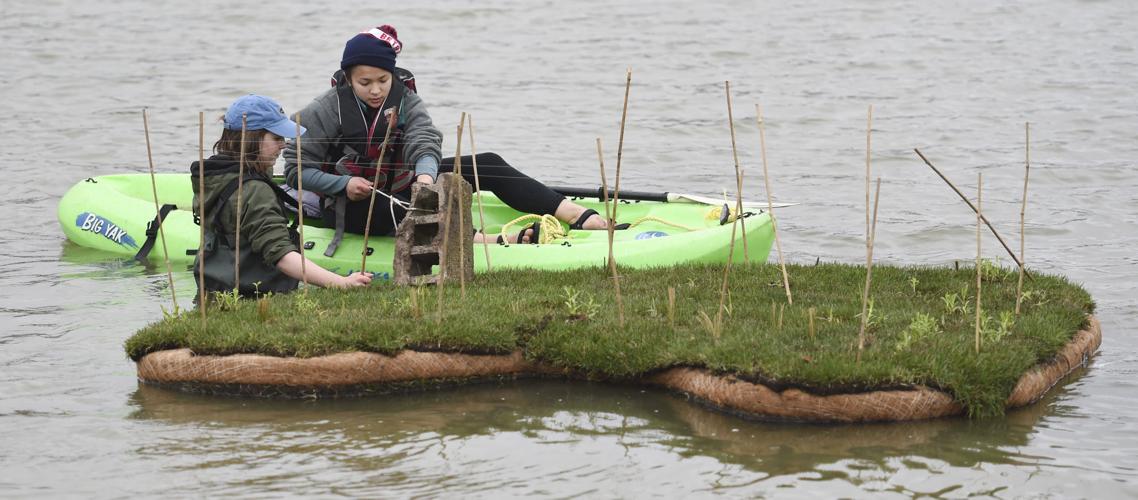The image depicts two young women engaged in an activity on a calm, shallow lake. One woman is seated in a bright green, sit-on-top kayak, while the other stands in the water up to her hips. Both women are dressed in warm clothing; the woman in the kayak wears a beanie and a gray shirt, while the woman in the water sports a blue baseball cap and a dark green sweatshirt. They appear to be working on a small, kidney-shaped floating grass island, not much bigger than the kayak. The island is adorned with several sticks protruding upwards, connected by wires at the top, and is populated with various plants, including bright green sprouts. A cinder block sits on the grass island, suggesting they may be tying something to it, possibly to anchor the island. The scene hints at a farming or scientific project, with the women focused on nurturing or structuring their floating garden in the glassy, blue-green water. The setting seems to be inspired by Thai or Filipino cultures, adding a layer of cultural context to their endeavor.